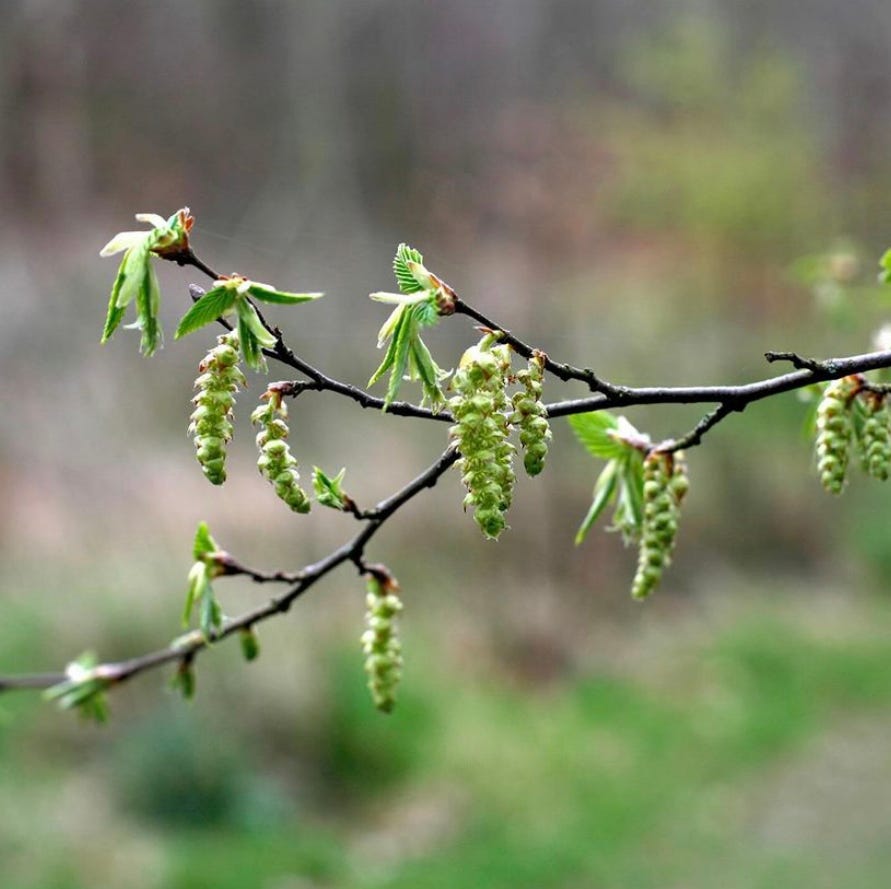This square-format color photograph captures a tree branch extending horizontally from the top right corner across most of the image. The branch divides into three larger segments from which several smaller branches sprout in both directions. Situated in an outdoor setting, the background is a blur of green and brown hues, suggestive of foliage and trees, contributing to the overall impression of early spring. The focal point of the image is the tree branch, adorned with about 10 green, acorn-shaped seed pods. These seed pods are elliptical and long, featuring small yellow hair-like structures at their ends. They hang down like tendrils from various spots where new buds are emerging. Surrounding the seed pods, clusters of green leaves are also sprouting. Despite the branch being the primary subject, it remains partially out of focus, especially towards its end, adding an artistic touch that emphasizes the natural beauty and detail of the budding leaves and seed pods against the blurred background.